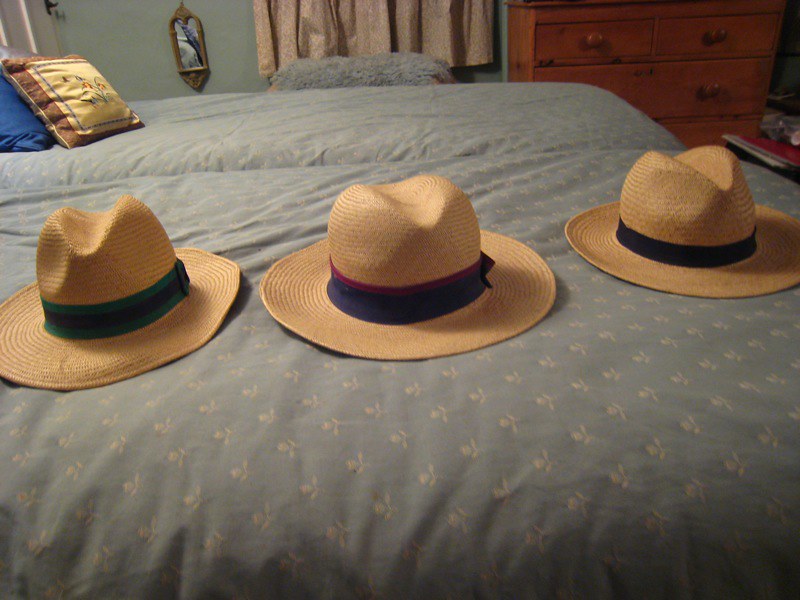The photograph depicts a cozy bedroom featuring two twin beds with matching light blue comforters adorned with a white single bud flower pattern. Centered on the bed closest to the viewer are three straw Panama hats aligned horizontally. Each hat flaunts distinct colored bands: the one on the left has a green band with a blue stripe, the middle one showcases a wide blue band with maroon trim, and the hat on the right has a simple black band. The beds have complementary pillows, with the front bed sporting a blue pillow under a brown pillow, which is highlighted with a blue outline and a floral motif. The room's walls are a teal color, complementing the light-colored curtains that can be partially seen alongside a wooden, oak dresser with visible brown knobs in the upper right corner. The overall atmosphere of the room is nostalgic and warmly inviting.